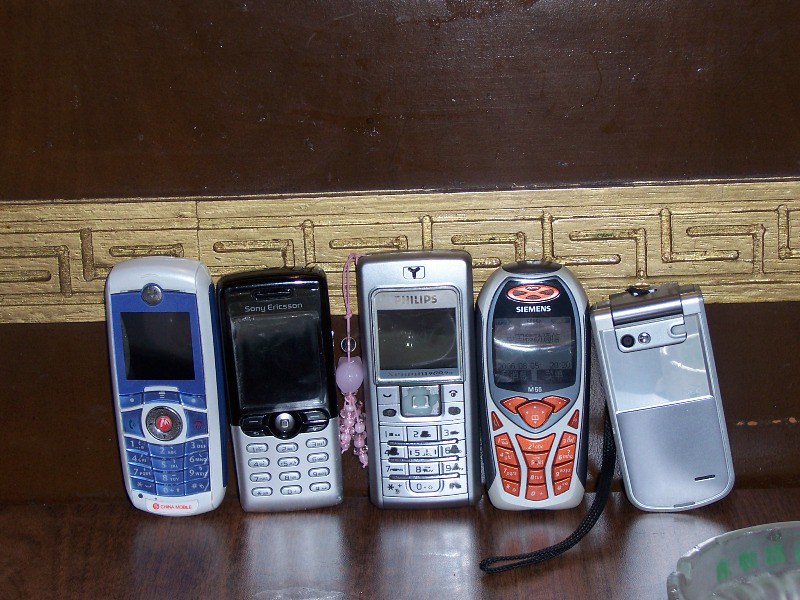A detailed photograph showcases a collection of five early 2000s cell phones meticulously arranged on a polished mahogany-colored surface. The bottom half of the image is dominated by this dark brown, reflective wooden table. Centered horizontally above the table is a strip of tan or gold wood, adorned with intricate, hieroglyphic-like carvings. Above this decorative strip, the wall continues in the same dark brown hue as the table, creating a cohesive backdrop.

From left to right, the first phone is a blue and silver rectangular device, identifiable by the faint emblem resembling Motorola's "M". Next to it stands a black and silver Sony Ericsson mobile, featuring a small screen and an older-style dial pad. The third phone, marked by the brand Philips, is predominantly silver with visible wear and tear, including faded markings and scratches, and it sports a pink charm that dangles from the side.

Following the Philips is a Siemens M55 model, distinguished by its gray body and orange buttons; it appears to be in the best condition among the collection. The final device, possibly a silver flip phone or a phone case due to its unusual clasp and black strap, faces backward, obscuring its keypad and making it difficult to identify the brand.

Additional details include a small, faintly visible green ashtray at the bottom right corner, notable for its cigarette indent. The overall scene is accentuated by the reflective quality of the wooden surface, capturing subtle reflections of the old, bulky cell phones that evoke a sense of nostalgia for the early era of mobile technology.